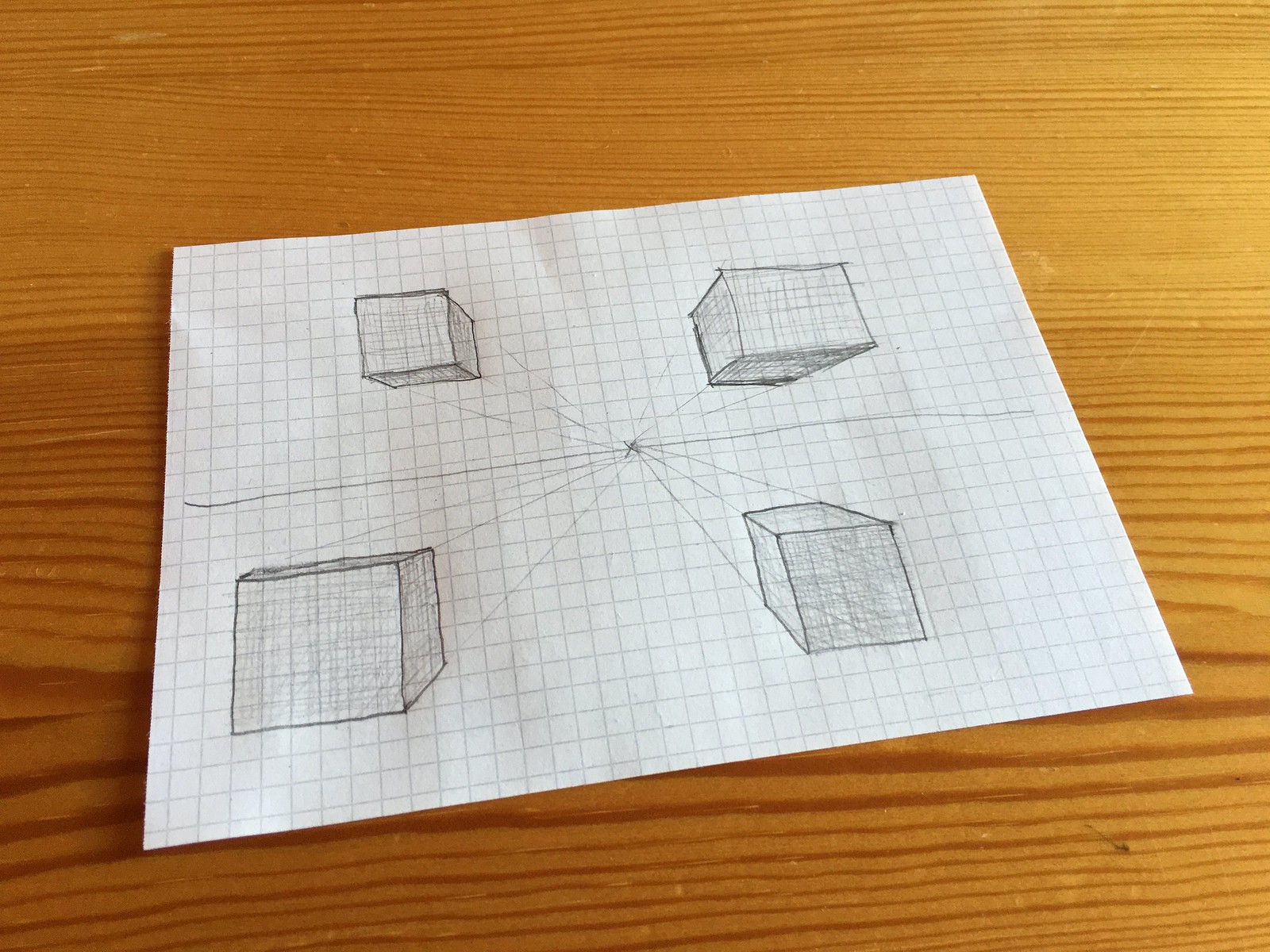On a rustic wooden table lies a white square piece of grid paper, diagonally oriented with the left edge positioned lower than the right. The grid is composed of light blue, small squares typical of standard graph paper. Dominating the visual composition is a horizontal pencil line that bisects the sheet. Each of the four corners is adorned with meticulously penciled, three-dimensional cubes, situated towards the center. At the very heart of the paper, a round, dark dot serves as a focal point, with pencil lines radiating from this central dot to each corner, connecting with the edges of the cubes.